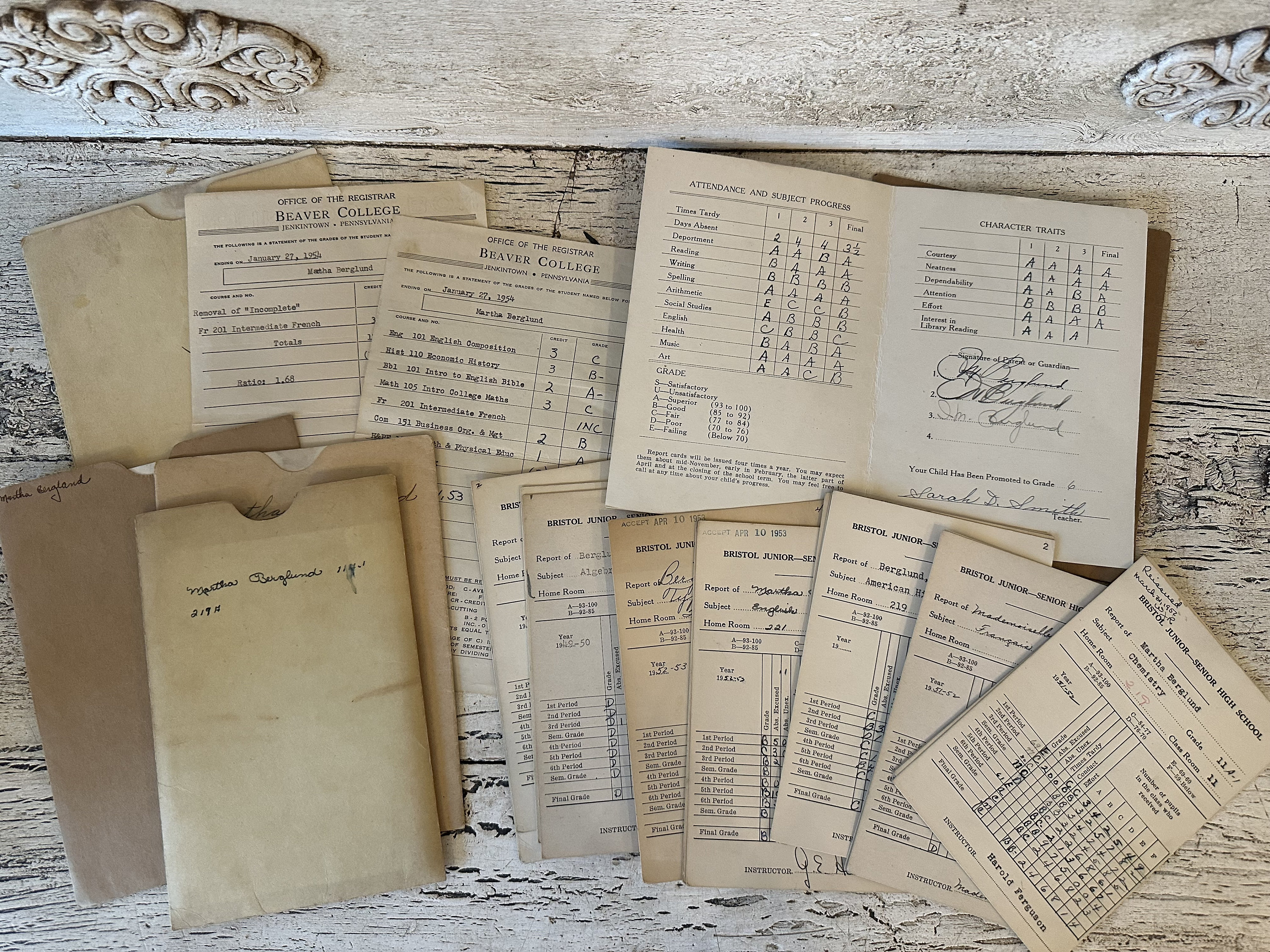The detailed image captures an antiqued, whitewashed wooden desk, characterized by its dark grayish-black crags and deep insets in the wood grain. The desk features elegant wooden filigree designs inset into the paneling at the top corners. Scattered across the desk are numerous weathered paper files that resemble old-time school report cards or transcripts. These papers are neatly arranged in folders with notched tops, primarily positioned on the far left of the desk. Many of the documents display official headings, such as "Office of the Registrar, Beaver College," accompanied by lists of grades, subjects, and attendance records. One visible open report card specifies details like classes on the left and grades on the right, with additional grades and signatures filling the opposite page. The report cards, which cover various educational details such as subject progress and character traits, prominently feature grade entries such as A's, B's, and C's, and span different quarters from Bristol Junior and Senior High School.